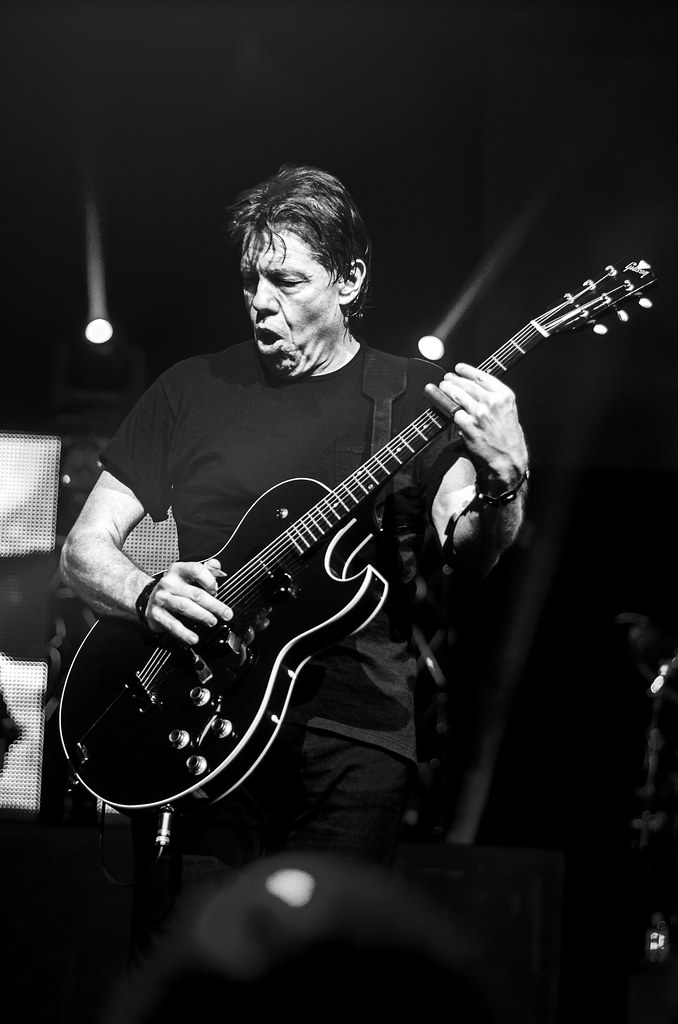This black-and-white concert photograph captures a mature musician on stage, playing an electric guitar with both hands while singing passionately into the microphone. Dressed in a black t-shirt and black pants, the musician’s short hair is flecked with silver, adding character to his stage presence. Behind him, two spotlights cast upward beams of light at 45-degree angles, illuminating the otherwise dark background. Further down, a black and white screen can be seen, contributing to the dramatic ambiance.